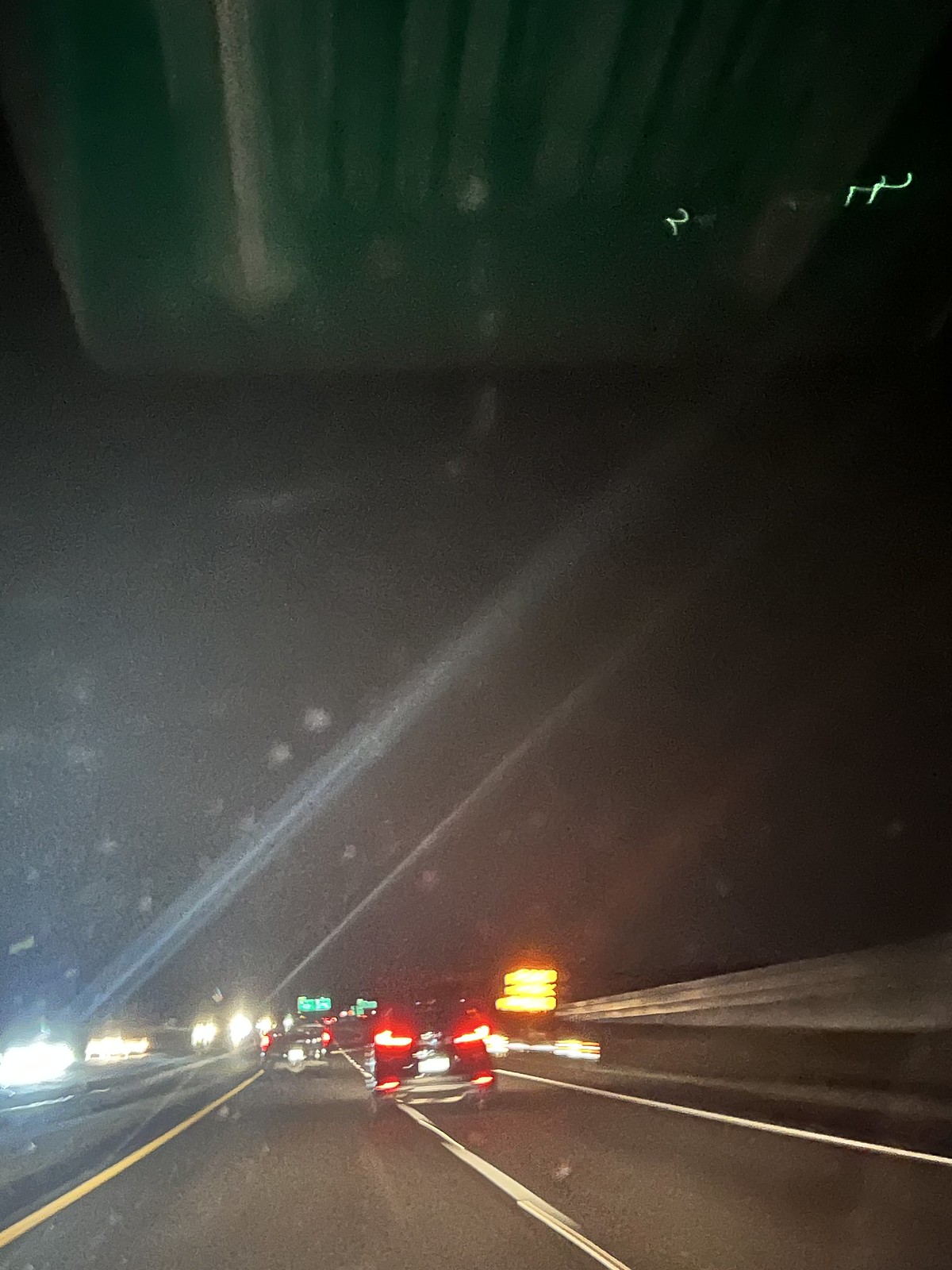This photograph captures a dynamic, night-time scene from the inside of a moving car. The image, taken through the windshield, features a highway bustling with activity. Directly ahead, a car is merging into the driver's lane, its red tail lights creating vivid, streaked patterns that accentuate the motion. On the left side of the scene, bright white lights from oncoming traffic shine intensely, separated by a glowing yellow dividing line. The road's white lines appear slightly blurred, further enhancing the sense of speed and movement. In the foreground, several green street signs offer a glimpse into the driver's journey, while the surrounding sky is filled with irregular blotches and streaks. These streaks appear to be reflections from the car's interior, adding an artistic, almost abstract quality to the photograph. Illuminated street or construction signs in the distance add additional layers and depth to this visually striking capture.